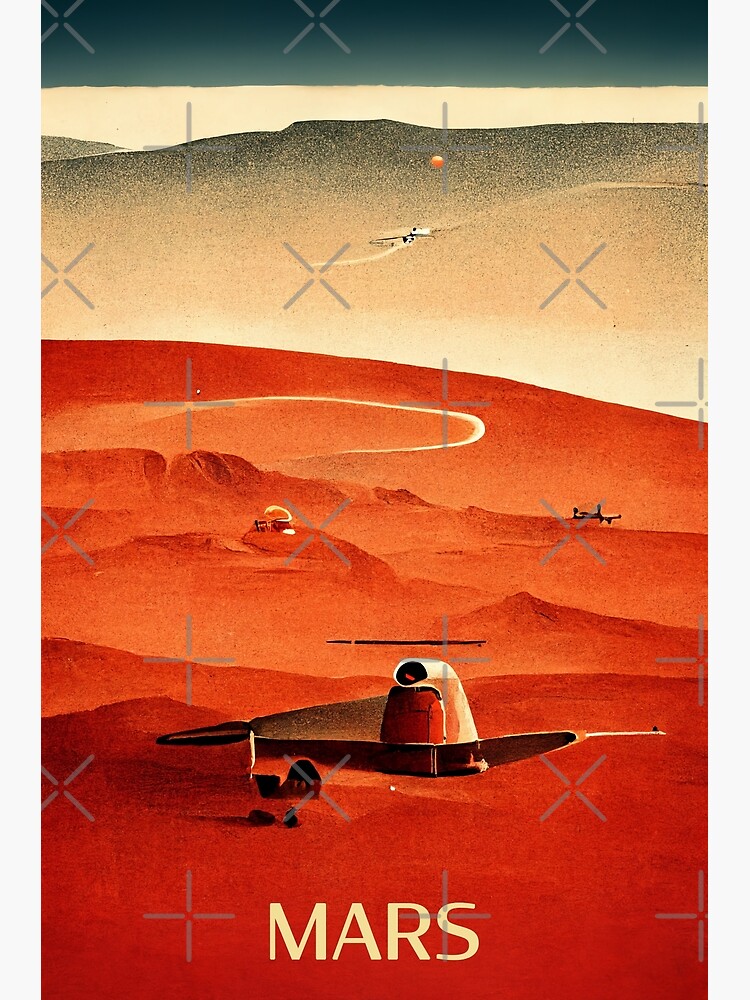The image depicts a vintage-style poster or book cover, prominently featuring a dramatic landscape of Mars. Dominating the lower half is a rugged, reddish-orange terrain interspersed with rocky formations and black-topped hills. A futuristic base with architectural elements resembling the 1970s sci-fi aesthetic is visible in the foreground. This base includes a saucer-like structure with a teacup-shaped dome, an exhaust vent, and an arched entrance carved out of the planet's red rocky surface. 

Above this base, the Martian surface continues with brown and red sand dunes populated with scattered steel towers. These structures appear to be part of the Martian settlement. In the background, a hazy white skyline blends into a dark turquoise greenish strip, creating a stark contrast against the planet's reddish hues. Further adding to the otherworldly ambiance, segmented gray X-shaped patterns are scattered across the skyline, each X featuring a central empty spot where its arms and legs meet.

At the bottom of the poster, the word "Mars" is prominently displayed in large, creamy beige lettering, underscoring the image's representation of a conceptual Martian landscape. This composition evokes the nostalgic charm of 1960s and 70s sci-fi book covers, offering a detailed and imaginative glimpse into human habitation on the Red Planet.